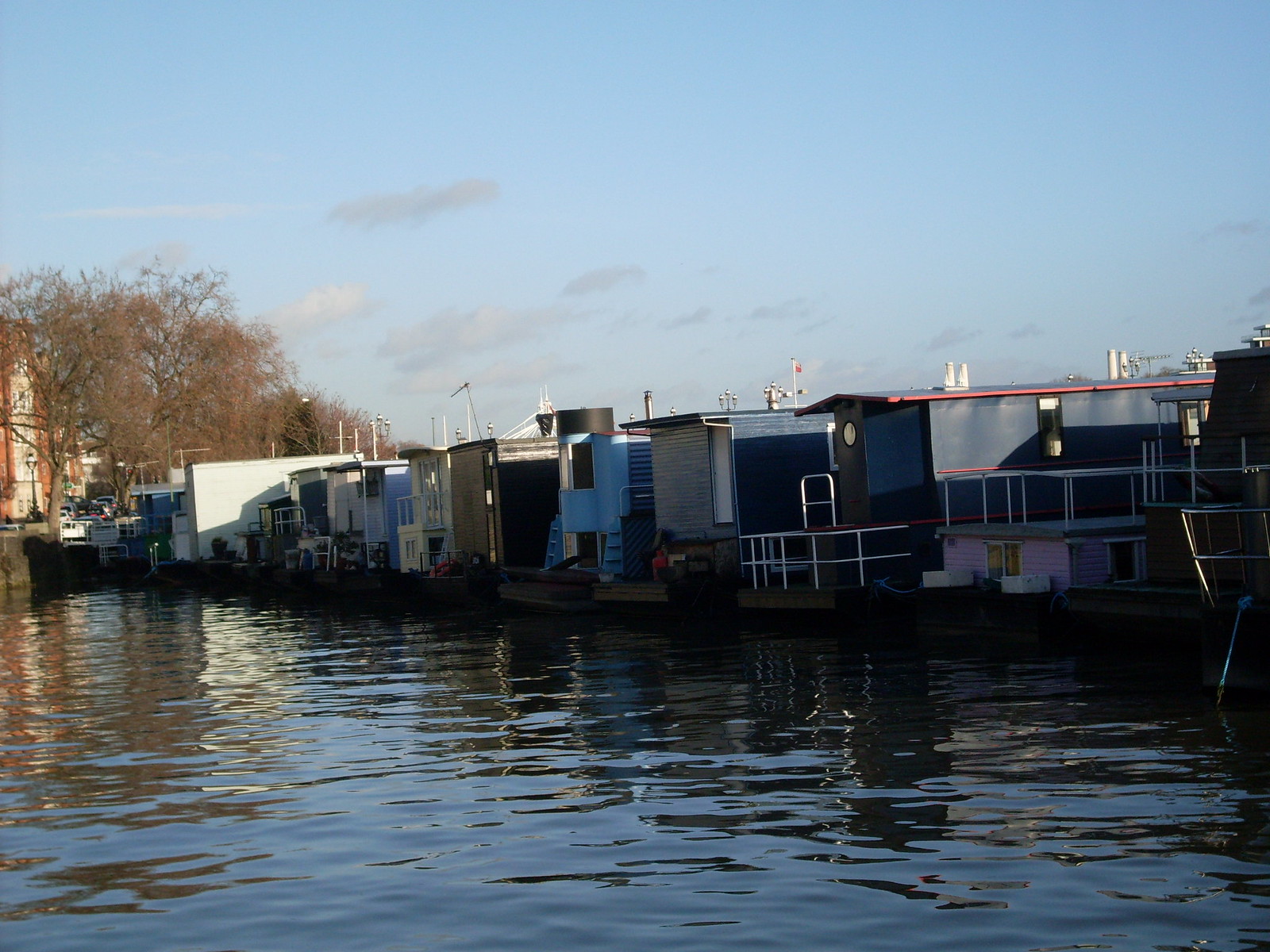A color photograph captures a tranquil waterway with dark, reflective water displaying gentle ripples and waves. The vivid image shows a cluster of houseboats, parked closely together, each with distinct designs and colors such as blue, red, light blue, dark blue, and white. These vessels give the impression of being somewhat ramshackle, similar to bait houses or shacks. Behind the water, densely packed buildings, resembling sheds or makeshift wooden structures, stretch from the center left to the center right of the image. To the left, thin trees with reddish berries or flowers stand out against the scene. A city street appears to cut diagonally across the background, lined with two-story brick and stone buildings. Above, the sky is a blend of light blue with patches of gray and white clouds. Some light reflects off the water, enhancing the calm and serene atmosphere of the scene.